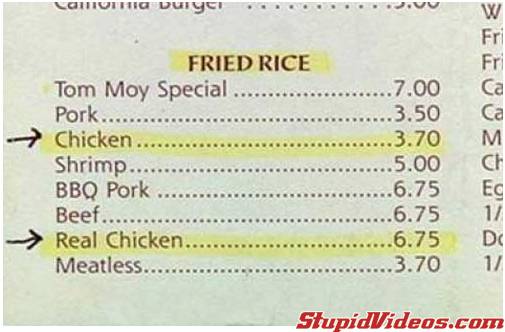The image is a grainy, close-up screenshot of a menu from a video hosted on stupidvideos.com. At the top of this menu, partially visible text suggests it may include items like "California Burger." The primary focus is on the "Fried Rice" section where various options are listed: Tom Moy Special for $7.00, pork for $3.50, chicken for $3.70 (highlighted in yellow with an arrow pointing to it), shrimp for $5.00, BBQ pork for $6.75, beef for $6.75, real chicken for $6.75 (also highlighted in yellow with an arrow pointing to it), and meatless for $3.70. The highlighted and arrow-marked differences between "chicken" at $3.70 and "real chicken" at $6.75 suggests a humorous discrepancy being pointed out. On the right side of the image, there is additional text in another column, though it is cut off and illegible. The watermark "stupidvideos.com" appears in red at the bottom left corner, indicating the image originates from an old online video.